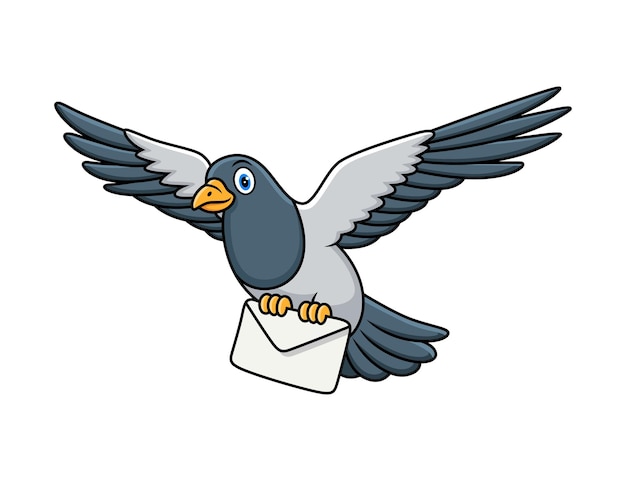This is a detailed digital illustration of a cartoonish homing pigeon, seemingly designed for children, with a vector-based minimalist style. The bird is depicted in mid-flight with its wings outstretched. It has a dark gray head, tail, and outer wing feathers, while the inner wing feathers and main body are light gray. Its bright blue eye stands out against its gray plumage and it has a thick, orange-yellow beak. The pigeon is facing left but appears to be looking directly at the viewer with a friendly expression. Its yellow clawed talons clutch a simple white envelope. The image lacks a background, featuring a plain white backdrop that emphasizes the pigeon.